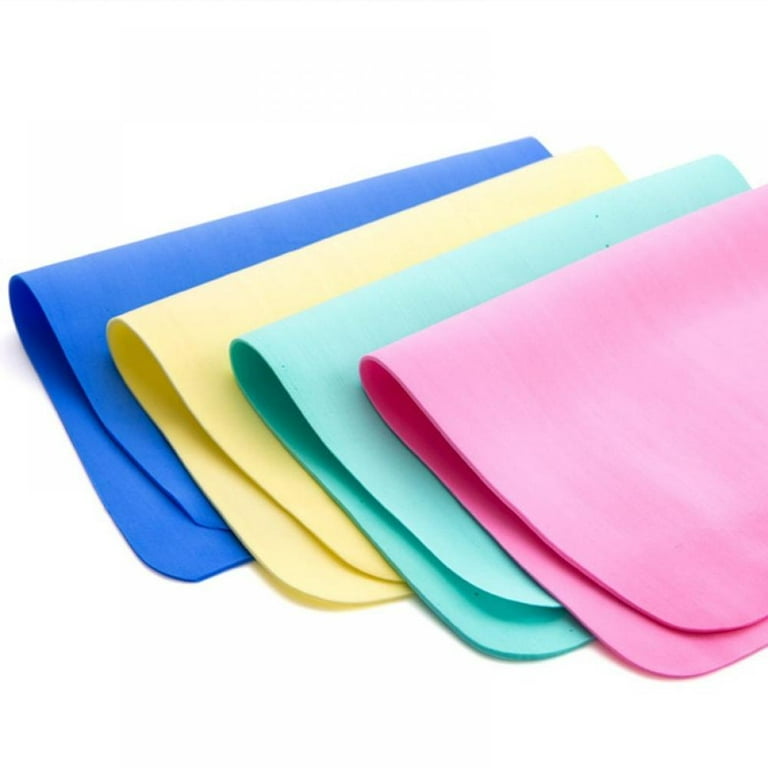The product photograph features four identical rectangular silicone mats, each in a different color: dark blue, yellow, light green, and pink. Each mat is folded halfway and stacked on top of each other, creating a layered pattern. The sequence from bottom to top is blue, yellow, light green, and pink. The background and surface of the image are edited to be completely white and void, ensuring the focus remains solely on the products. Notably, the light green mat features small indents or holes near the top section. The photograph, designed for online shops, websites, or catalogs, presents a square composition with all four sides of the image being equal in length. The mats are thin, flexible, and exhibited in a way that only partial views of each are visible due to the overlapping arrangement.